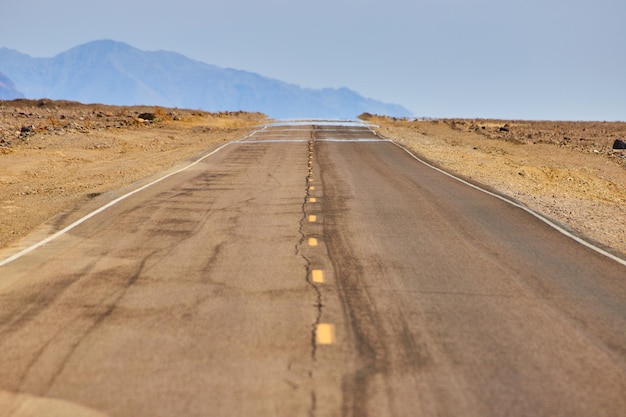The image captures a desolate highway stretching through what appears to be a desert landscape, most likely in the southwestern United States, such as New Mexico or Arizona. The black paved road, showing signs of wear with numerous cracks and marks, extends straight into the distance, where it appears to vanish into a hazy point at the horizon. Running down the center of the highway are dashed yellow lines forming a V-shape perspective. On either side of the road, the ground is a barren mix of tan and gray sand interspersed with scattered gray and black rocks, emphasizing the harsh desert environment. The scene is set under a clear, sunny sky devoid of clouds, enhancing the mirage effect of water on the distant asphalt. In the far background, the faint outlines of mountains, slightly darker in blue, can be seen blending into the horizon, adding depth to the expansive and arid atmosphere of the image.